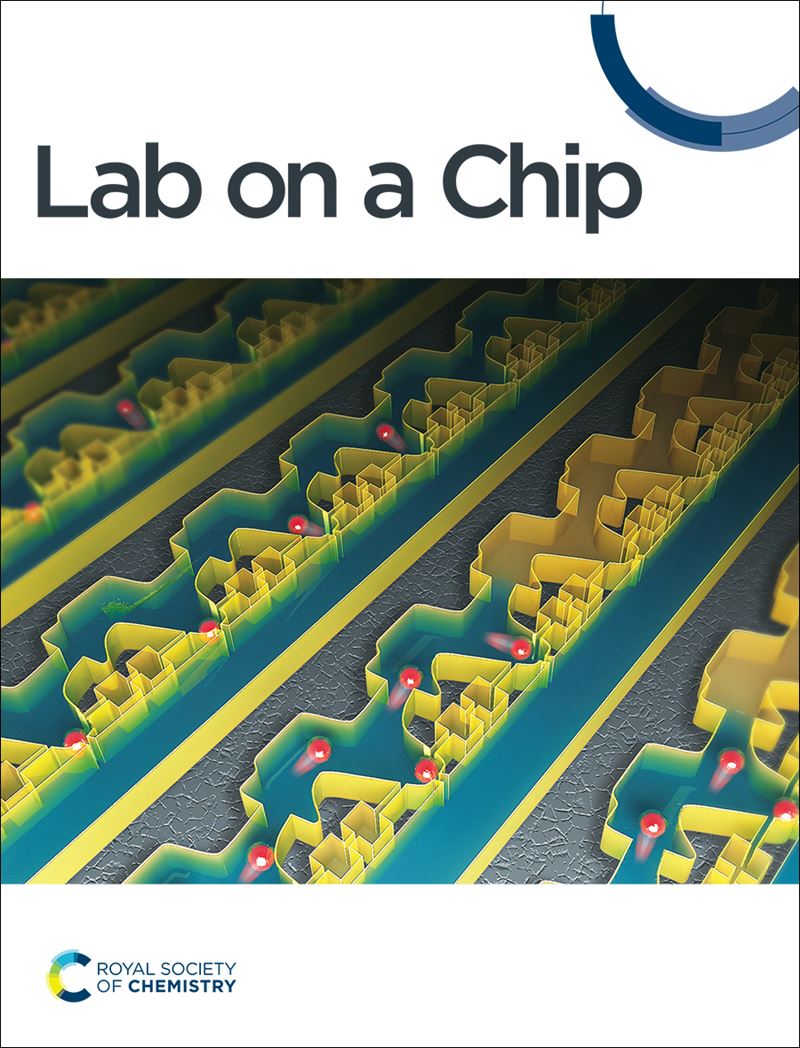The image is a cover, possibly of a poster, flyer, or booklet, depicting an abstract, computer-generated artwork. It is divided into three sections. The top section features a white header with the title "Lab on a Chip" in black text. In the upper right corner of this header, there is a semi-circle formed by thick, blue lines. Below the header is the central section, a visually complex and colorful depiction that might represent the inner workings of a computer chip or microscopic chemical processes. This section includes multiple yellow shapes filled with green liquid, interspersed with curved, wrinkled, gray surfaces. Scattered throughout these yellow shapes are numerous red balls that appear to be bouncing or moving. The artwork evokes a sense of magnified detail and intricate pathways, akin to chemistry or lab processes. The bottom section of the cover is another white banner, displaying the text "Royal Society of Chemistry" in blue, alongside a multicolored 'C' logo, which includes shades of black, blue, yellow, and another black section. The cover is bordered by a thin black line, giving it a clean, framed appearance.